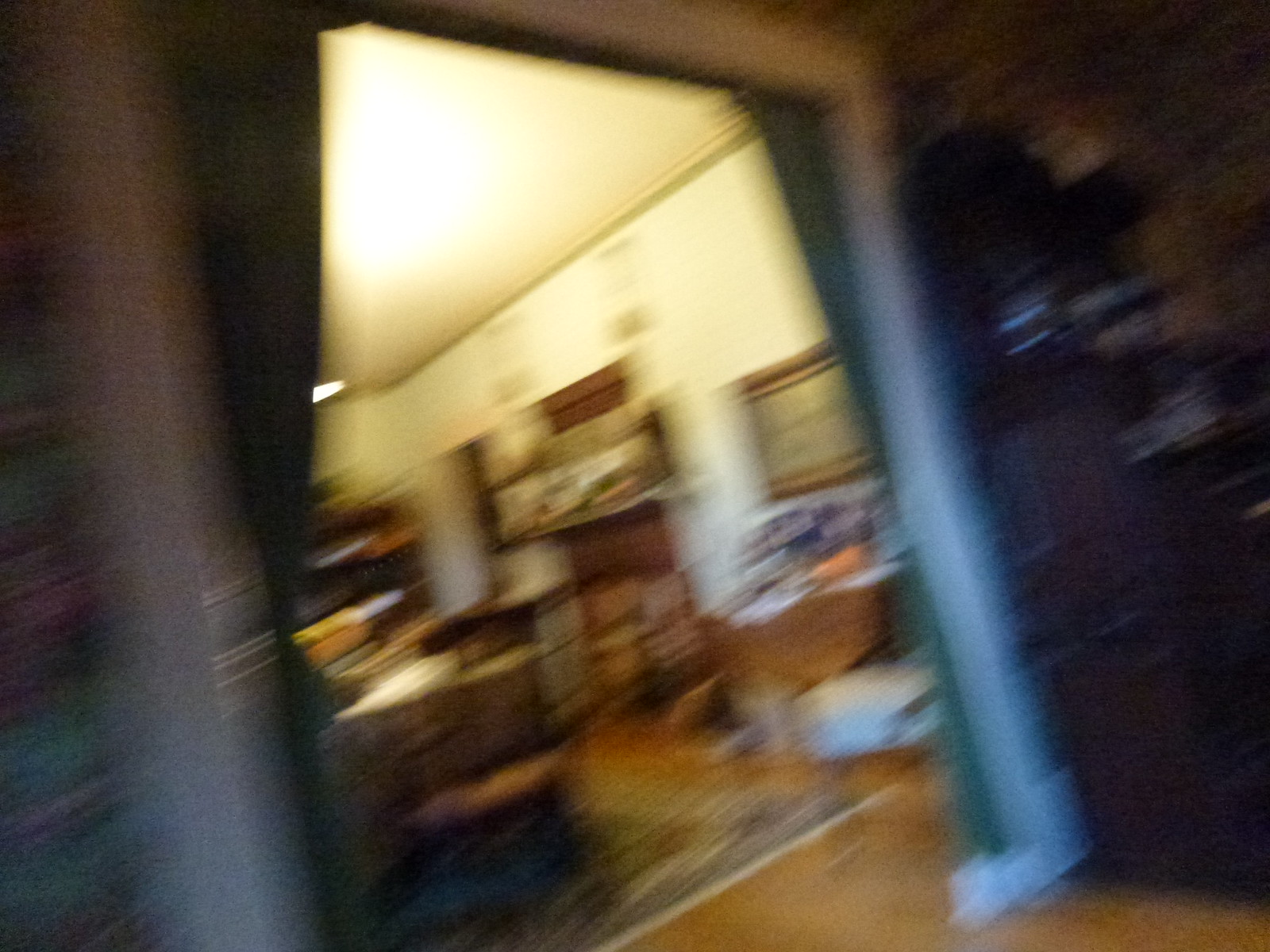The image depicts a very blurry interior of a home, looking from a darkened room into a well-lit living room. Visible through a white-bordered entryway, the living room is filled with assorted items, almost resembling a mini hoarder's space. A bright ceiling light illuminates the room, casting a yellow hue over the scene. Though it’s difficult to make out details due to the motion blur, there are several brown tables cluttered with papers and various items, including discernible orange and yellow objects. The floor appears to be wooden, partially covered by a rug, and brown chairs can be seen underneath some tables. Additionally, the white walls are adorned with numerous pictures, one of which is framed in brown. Flanking the entryway are dark green curtains, adding to the sense of peering into the luminous, cluttered room from a darker space.